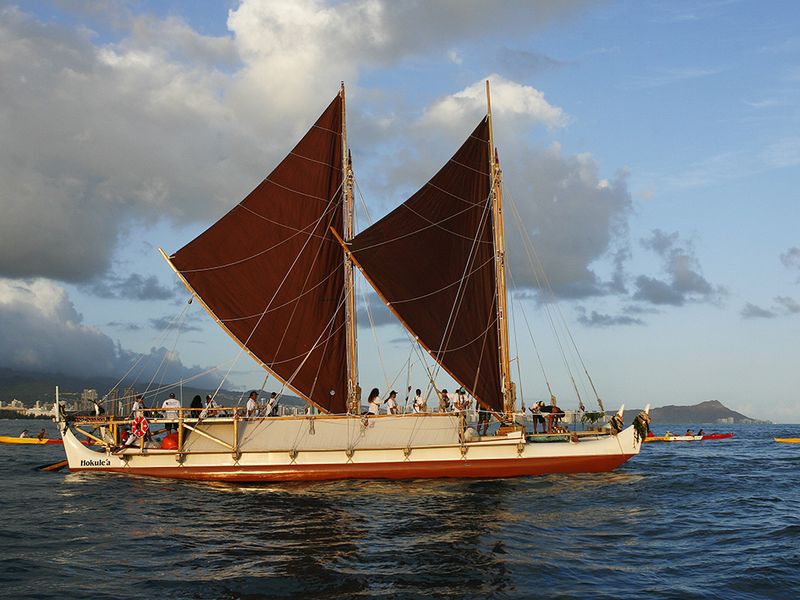In this image, a striking sailboat named Hokulea, identifiable by the name inscribed on its side, sails through vibrant blue waters. This sailboat is designed like a catamaran, resembling two long canoes with a white top and a brown underside that delves into the water. The boat boasts two masts with triangular, maroon sails supported by ropes. Around 15 people are visible onboard, actively engaged in various activities. The scene is set against a backdrop of a mountainous island, likely the Hawaiian coastline, with dark gray clouds hovering over the peaks on the upper left side. The rest of the sky is an expansive blue with a few light clouds scattered. The foreground of the image includes several kayak boats manned by paddlers, enhancing the dynamic feel of this daytime nautical scene. Far in the distance to the left, the silhouette of large buildings, potentially from Honolulu, can be seen, providing a subtle urban contrast to the natural beauty surrounding the sailboat.